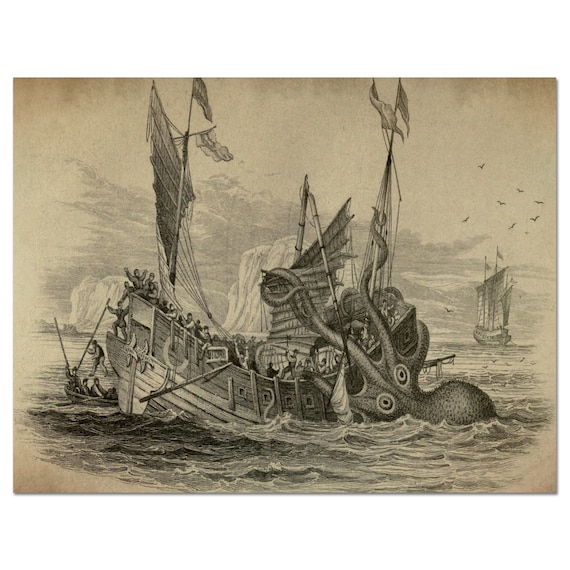This detailed, old-fashioned black-and-white sketch, possibly from an ancient book, depicts a dramatic maritime scene with a striking sense of age evident in the faded canvas edges. At the forefront, a 17th-century-style sailing ship, likely a galleon with two large wooden masts, is under vicious attack by an enormous kraken or giant squid. The creature's powerful tentacles emerge from the water, gripping the ship and its sails, causing significant distress among the potentially hundreds of sailors depicted onboard. The main mast of the ship, now severed, is collapsing into the ocean as some sailors desperately flee into a smaller lifeboat. Behind the besieged vessel, another sturdier ship stands in the distance to the right, more heavily rigged and capable, but not currently involved in the chaos. Adding to the scene's authenticity, sea birds hover above, and two large icebergs loom in the background, contributing to the overall sense of peril and urgency.